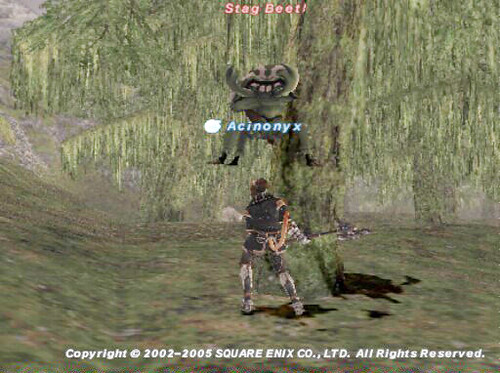This still image appears to be from an animation, possibly from the EO game. The animation quality is grainy, and the resolution is not very high. The scene captures a grass surface that displays a spectrum of green, interspersed with varying shades of light and dark brown. A prominent willow tree stands at the center, characterized by its thick, dark brown trunk adorned with greenish moss. The tree's branches are large, with leafy tendrils hanging down. In front of the tree, a character clad in what resembles tactical gear is standing. At the top of the image, "Stag Beetle" is inscribed in red letters, accompanied by an image of a beetle labeled "Xenonix." Below this, in white text, it reads, "Copyright 2002-2005, Square Enix Co., Ltd., All Rights Reserved."